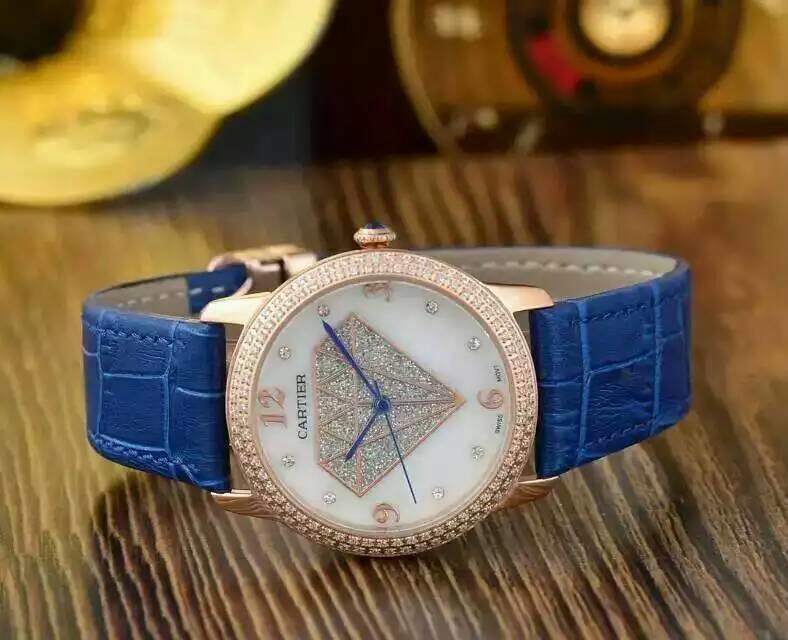The image features a luxurious wristwatch elegantly displayed on a richly textured, brown wooden surface with pronounced wood grain patterns. In the background, there are several indistinct items, giving a subtle depth to the composition. On the right side, a circular object with a brownish hue and touches of red is partially visible, while on the left side, another light yellowish circular item can be seen.

The wristwatch itself boasts a sophisticated blue leather strap. Its circular watch face is framed by a border encrusted with what appears to be diamonds. The pristine white watch face features a prominent diamond shape, seemingly composed of smaller diamonds, adding to its opulent design. There are four key numerical markers in striking pink: 12, 3, 6, and 9. The positions of the remaining numbers are marked by small circular diamonds.

Between the 12 o’clock position and the central diamond shape, the prestigious brand name "Cartier" is displayed. The watch hands, colored in a refined blue, elegantly indicate the time, which reads 10:09 and approximately 43 seconds. The hour, minute, and second hands add a final touch of precision to this exquisite timepiece.